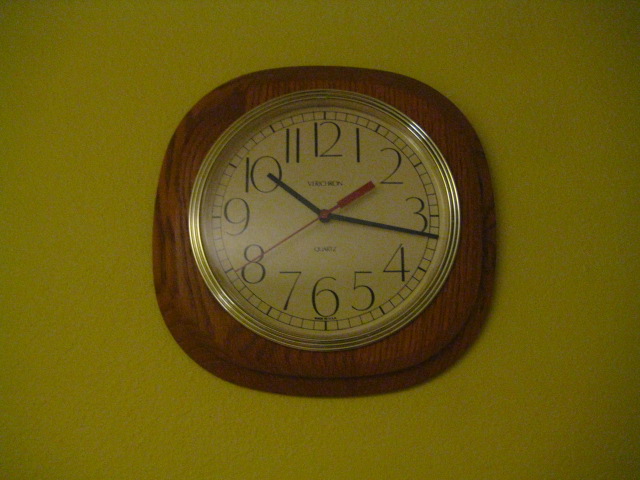A meticulously crafted wooden wall clock is displayed prominently against a pea green wall. The clock boasts a robust wooden frame, exuding a sense of sturdy elegance. Encircling the face of the clock is a gleaming gold border, adding a touch of sophistication. The clock face is an ivory hue, rich and warm, complementing the earthy tones of the wood and gold. Large black numerals stand out clearly against the ivory background, with fine lines denoting each minute and hour around the circumference. The time reads 10:16, with the slender minute and hour hands elegantly pointing to their respective positions. A striking red seconds hand, meanwhile, is paused at the 8, providing a vibrant contrast against the subdued palette.